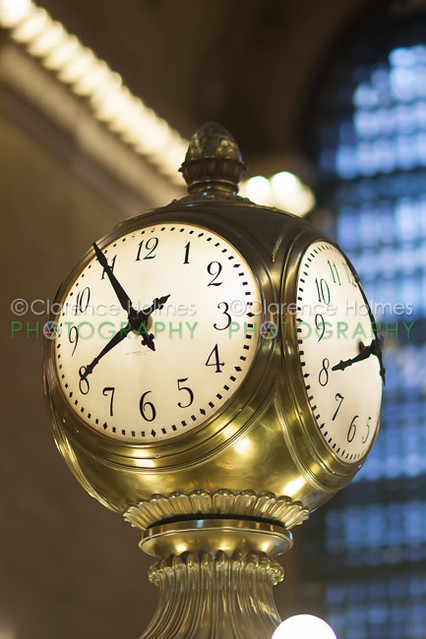This photograph captures a stunning four-sided clock prominently situated in what appears to be a terminal. The image, branded with "Artistic Photography" across the top, highlights the elegance of the clock’s design. Two of the clock faces are clearly visible, showcasing rounded, white backgrounds with bold black numerals. The current time reads 7:55, with metal hands indicating the hour and minute. The clock is encased in polished brass, exuding an air of sophistication and vintage charm. Atop the clock sits a rounded finial, supported by a meticulously scalloped neck that transitions seamlessly into a straight section before continuing its scalloped design downward. The backdrop boasts a large privacy-glass window, adding to the ambient lighting of the scene. String lights drape elegantly against a brown wall, accentuating the clock's timeless beauty and the terminal's inviting atmosphere.